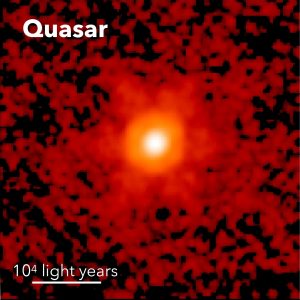The image is a long-distance photograph of a quasar, captured through a telescope, depicting a complex and mesmerizing celestial phenomenon. In the center of the square image, a bright, white circle is prominently featured, representing the highly luminous core of the quasar. This central white circle is encased within an orange ring, which itself is enveloped by a fiery, six-pointed star pattern. Surrounding this central formation are multiple red and dark red dots, interspersed with black dots, creating a textured effect against the primarily black background. The intricately detailed image is accentuated with white text in the top left corner that spells "QUASAR" and in the bottom left corner, the text "10^4 light years" appears above a white line, indicating the distance of the quasar from Earth.